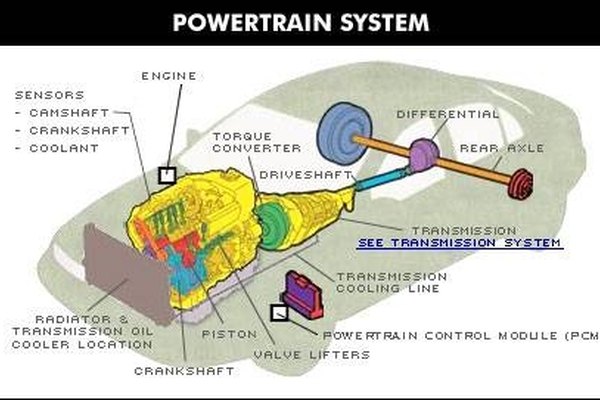The image is a technical illustration of a car's inner workings, specifically focusing on the Powertrain System. At the top of the diagram, the words "Powertrain System" are displayed in bold white text within a long, thin, horizontal black rectangle. Beneath this, a grayish-tan drawing of a car occupies the center of the image. Superimposed on the car are various color-coded components of the Powertrain System, each element clearly labeled with black arrows pointing to them.

The engine, prominently shown in yellow, has detailed internal parts depicted in different colors: a red piston, a light blue crankshaft, and green components representing the torque converter. The driveshaft is colored in blue, while the differential at the rear axle is highlighted in purple. The radiator, placed towards the front of the car, is shown in a darker gray.

Surrounding the car's schematic are labels and annotations identifying additional parts, such as the camshaft, valve lifters, sensors, coolant, transmission oil cooler location, powertrain control module (PCM), and transmission system. Orange bars indicate the positions of the rear axles. The illustration is akin to an anatomical diagram, meticulously mapping out the intricate details of a car's Powertrain System, offering a comprehensive overview of its components and their placements.